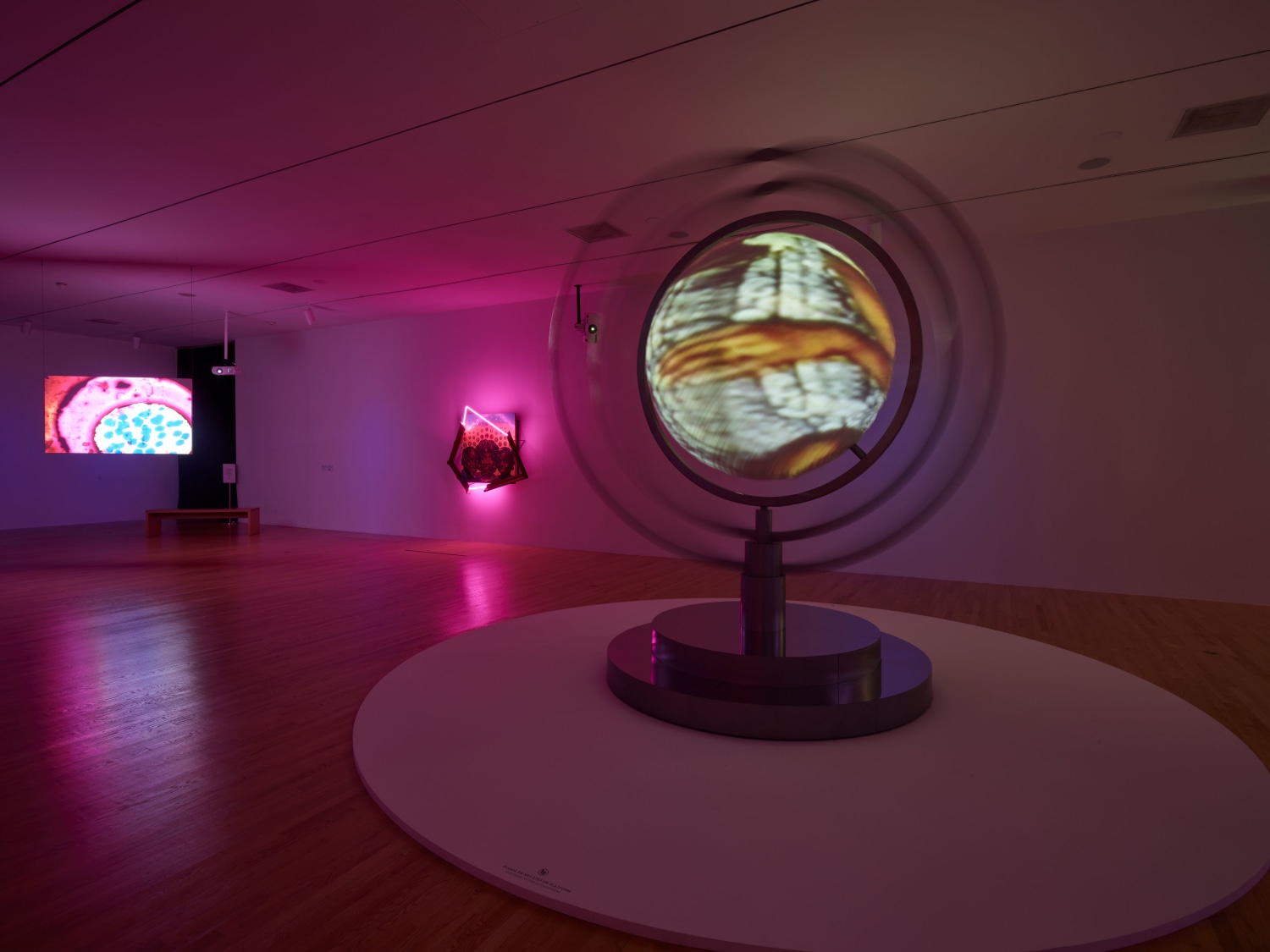The photograph, taken in landscape orientation, captures the interior of a large, mostly empty room with light pink walls and ceiling. The floor is composed of medium brown hardwood. In the center of the room, there are two stacked circular platforms: a larger white one on the bottom and a smaller dark brown or black one on top. On the upper platform, an intricate object stands out, consisting of a globe with various circular rings encircling it. This globe, unlike a traditional earth globe, features light gray and brown hues.

On the right side of the floor, another globe can be spotted, though it lacks the circular rings. Adding to the room's minimalistic decor, a display screen or monitor hangs on the far left wall, emitting vibrant blue, pink, purple, and red colors. The room is dimly lit, with colored lights enhancing certain elements such as the aforementioned rings, giving the impression of motion. Additionally, the front wall features several design paintings, from which unique light patterns emanate.